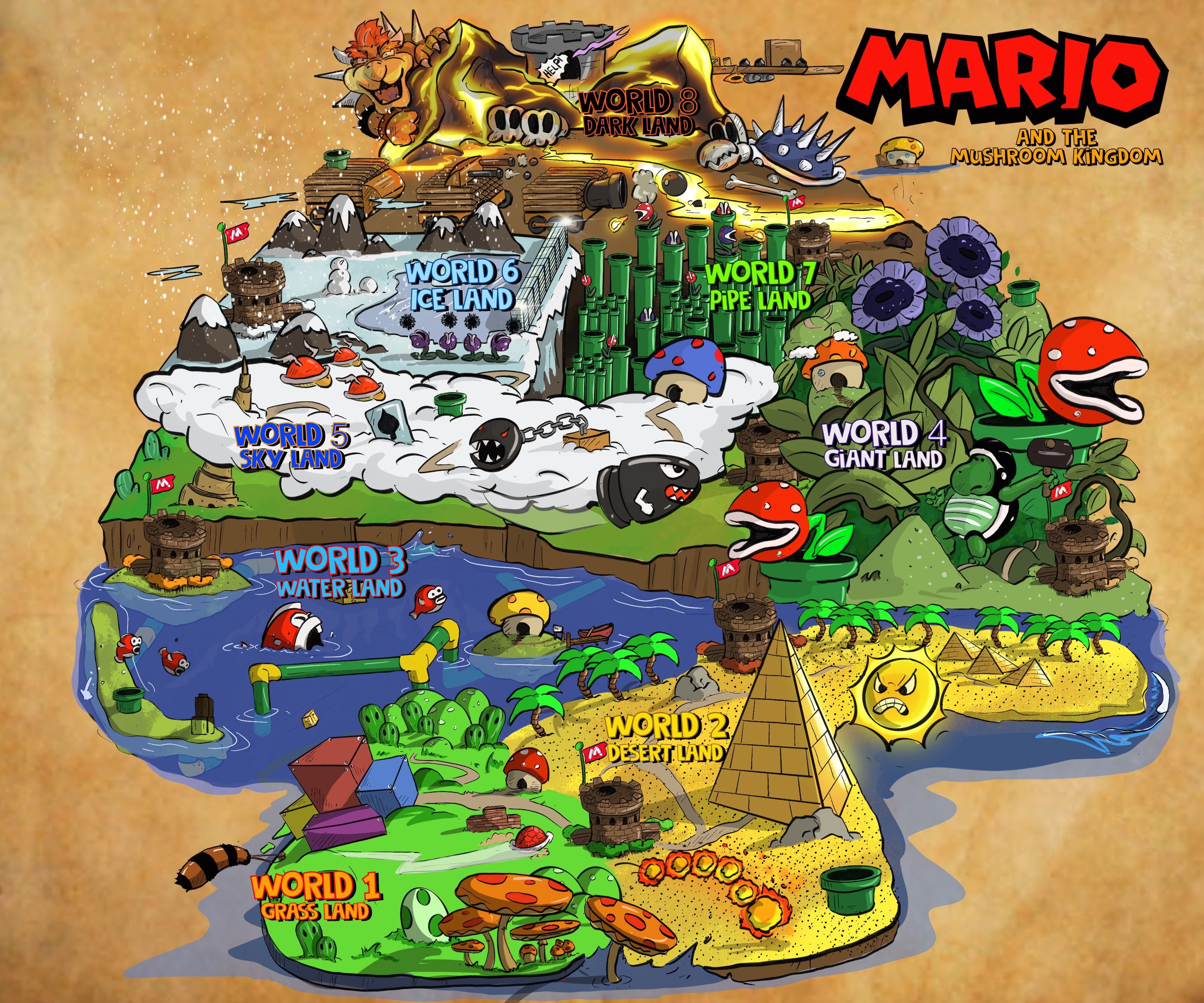This image is a detailed, colorful map of Mario and the Mushroom Kingdom, shown in a cartoon-like style with vibrant depictions of various worlds and traditional Nintendo elements. In the upper right corner, "Mario and the Mushroom Kingdom" is prominently displayed in bold, traditional Nintendo font. The map represents an overworld layout starting from the bottom left and moving upward.

At the bottom left is World 1: Grassland, highlighted in orange text. This area features a grassy landscape with large mushroom stalks that are orange at the top with red dots, and a white Yoshi egg with green spots. Various colored blocks and mushroom houses are also visible.

Moving right, we encounter World 2: Desert Land. This section is characterized by traditional Mario and Nintendo enemies, including the fire caterpillar and the iconic green pipe. A pyramid, desert palm trees, and the menacing angry sun emphasize the arid environment.

To the left of Desert Land is World 3: Waterland, labeled in blue text. This aquatic world showcases the classic Mario fish enemy—a red fish with white lips—alongside more green pipes and a yellow mushroom house.

At the very right is World 4: Giant Land, where everything is markedly larger. Giant piranha plants tower over the landscape, accompanied by another mushroom house and various oversized flowers. A green Koopa, a helmeted turtle-like enemy, can be spotted here.

Proceeding leftwards, World 5: Skyland appears as a cloudy environment. Iconic Mario enemies such as the Chain Chomp and Bullet Bill inhabit this lofty world.

Above Skyland lies World 6: Iceland, filled with icy, snow-covered terrain.

To the right of Iceland is World 7: Pipeland, a domain dominated by a multitude of green pipes, representing the intricate network of tunnels familiar to Mario players.

At the very top of the map is World 8: Dark Land, Bowser’s sinister territory. Bowser can be seen peeking from behind a mountain, with his ominous castle adorned with skulls in the background. This is the final and most daunting world, where the ultimate challenge awaits.

Together, these detailed elements create a vivid and comprehensive depiction of Mario and the Mushroom Kingdom, inviting the viewer into the diverse and adventurous world of Mario.